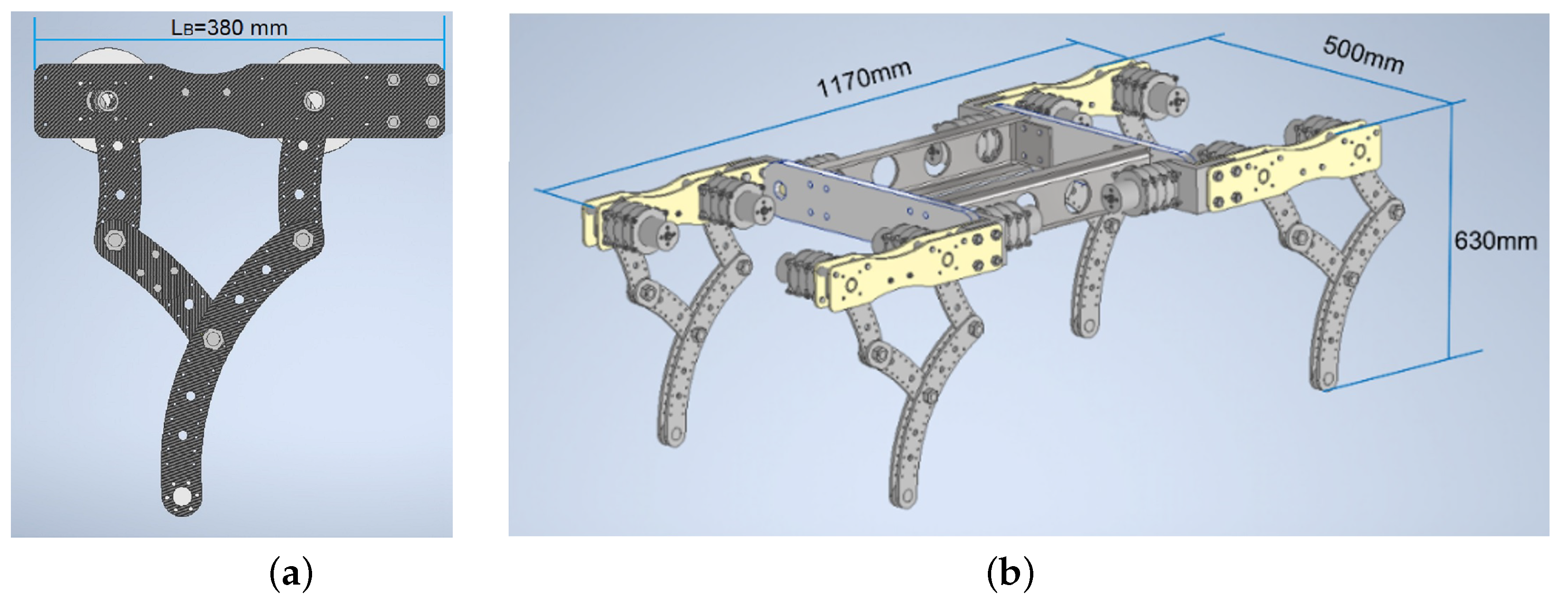The image is a detailed, computer-generated diagram used to illustrate measurements and assembly instructions, featuring a light blue background. The diagram is divided into two sections, labeled as Diagram A and Diagram B, positioned side by side. 

Diagram A showcases a side view of a metallic piece, likely a part of a robotic arm or a metal stand, connected by several screws. This piece is labeled with the measurement "380 millimeters" in black lettering at the top, accompanied by the letter 'A' underneath.

Diagram B presents a more complex structure that appears to be an entire assembly, possibly a robotic rover with multiple armatures. The assembly includes eight electric motors and demonstrates a complete setup where these motors control the movement of the armatures, which act as legs for the robot. The dimensions of the entire assembly are prominently displayed as 1,170 millimeters in length, 500 millimeters in width, and 630 millimeters in height, with the label 'B' underneath.

The image's color scheme mainly includes shades of gray and light yellow for the metallic parts, with the text and measurement indicators in black. The detailed labeled measurements and components resemble what one might find in a technical manual or a construction guide for precise assembly.